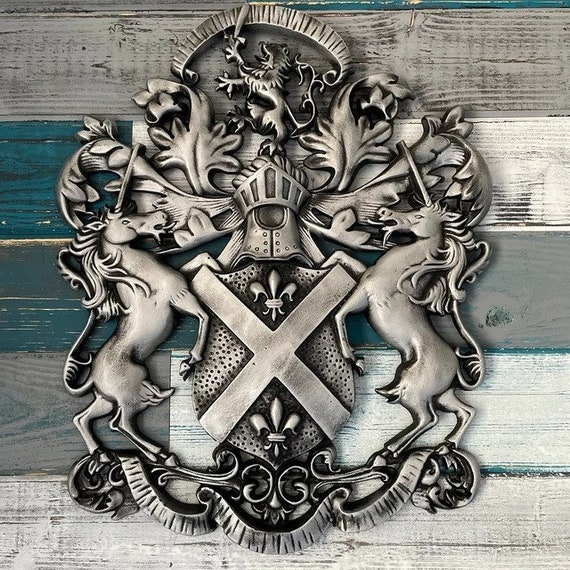The image depicts a highly intricate silver family crest mounted on a weathered wooden background composed of horizontal planks painted in alternating shades of blue, gray, and white. Central to the composition is a large shield adorned with a prominent X and two fleur-de-lis, one above and one below the X. Flanking the shield are two unicorns standing on their hind legs, each facing inward with their front legs raised. Above the shield sits a detailed medieval knight’s helmet topped with a crown. Crowning the entire crest is a lion-like creature standing on one leg and brandishing a sword. The ornate design is enriched with decorative leaf and scroll patterns that weave around the central elements, encapsulating the entire artwork with additional filigree. The crest rests flat against the planked background, its burnished silver surface displaying a patina that highlights the fine details of the craftsmanship. At the very bottom, a ribbon-like banner completes the composition.